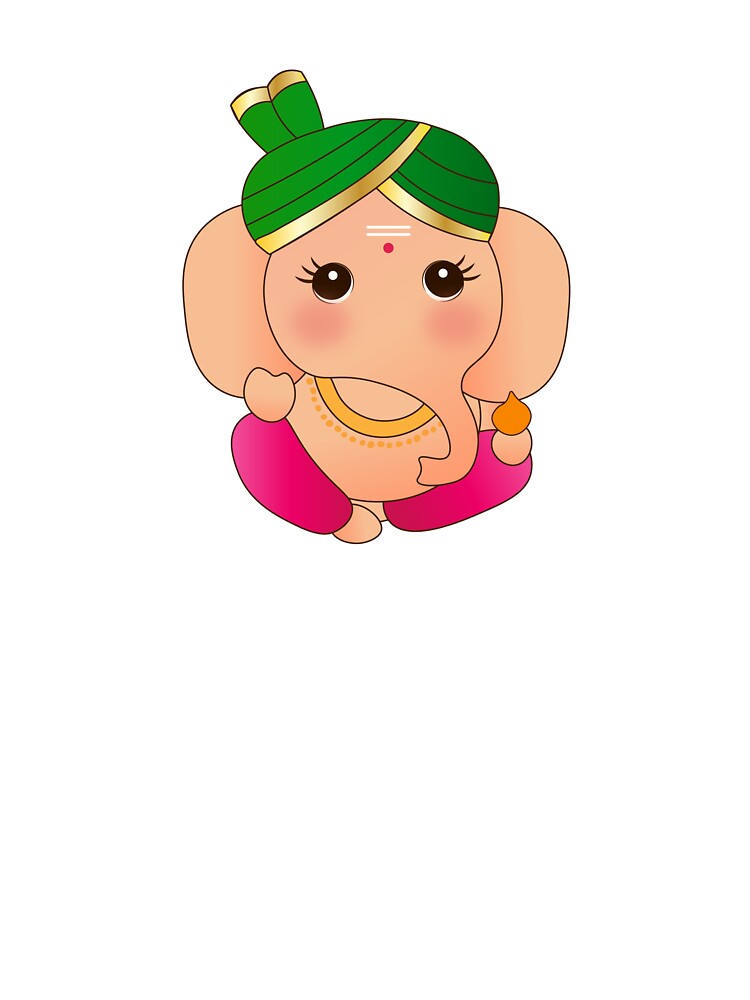This image is a simple, yet detailed cartoon illustration of a meditating elephant. The elephant's body is a peach-pink color, with large, expressive brown eyes adorned with three lashes each, against a backdrop of blush beneath them, creating a sad, gloomy look. It lacks a nose and mouth, featuring only a trunk that hangs down towards its belly. The elephant is adorned with a bright green turban decorated with gold iridescent trim, and a prominent ruby-like red dot centered on its forehead, accompanied by two horizontal white lines above it, indicating an Indian cultural influence.

The elephant is dressed in a green tunic with gold borders, paired with pink to magenta pants, with its small, round feet emerging from the bottom. It sits in a nearly lotus position, with each hand resting on its respective knee, holding an inverted peach-shaped orange object in its left hand. Around its neck is a gold chain and an orange Indian-style necklace. The large pink ears and cheeks enhance the cute and cartoonish aesthetic of the figure.